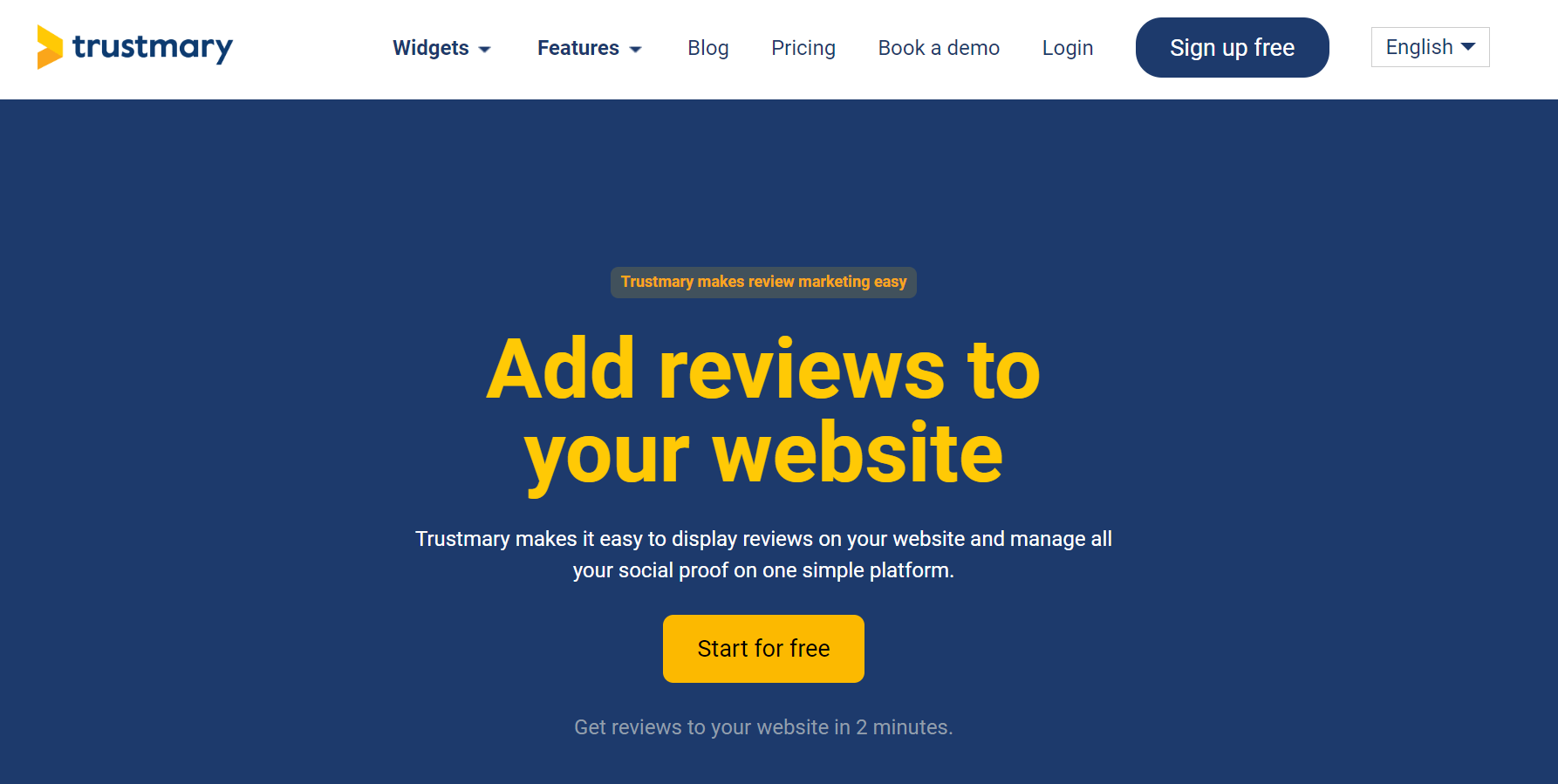The image features a prominently branded header with "Trust Mary" displayed in the top left corner, accompanied by a small yellow logo resembling a sideways "V" pointing to the left. Adjacent to the logo are various menu categories including "Widgets" and "Features" in dark blue, followed by "Blog," "Pricing," "Book a Demo," and "Login." Further to the right, a bubble-shaped element highlights the option to "Sign Up for Free," while the top right corner features a rectangular box with the language selection, labeled "English."

Dominating the center of the image are the prominent phrases designed to attract attention. At the top, "Trust Mary makes review marketing easy" is written in vibrant orange text. Below it, "Add reviews to your website" stands out in bold yellow text. An explanatory line underneath states, "Trust Mary makes it easy to display reviews on your website and manage all your social proof on one simple platform," rendered in crisp white text. 

At the bottom middle, there is a call-to-action button in a square box labeled "Start for Free," with an orange background and black text. Finally, the footer contains a concluding message, "Get reviews to your website in two minutes," emphasizing the platform's efficiency.

This detailed composition emphasizes Trust Mary's capabilities in facilitating review management and marketing on user websites, presented in a visually appealing arrangement with strategic use of color and text positioning.